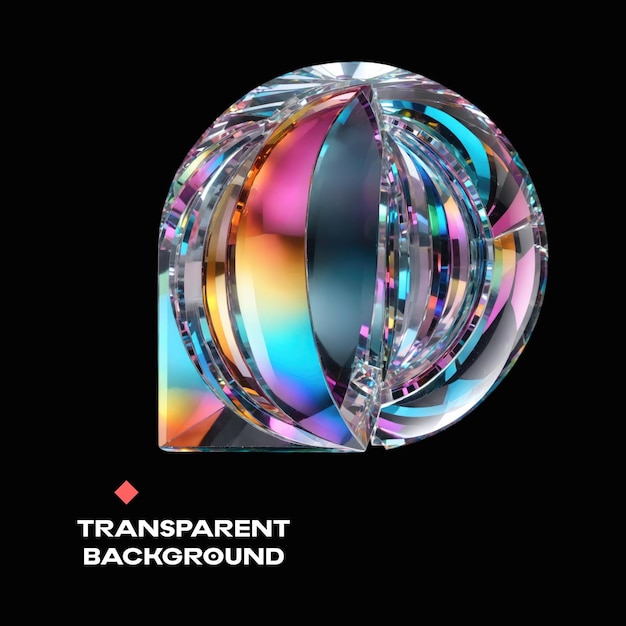Set against a solid black background, this image features a central giant circle reminiscent of a disco ball. The circle is segmented into various colors, with the front section prominently displaying pink, yellow, teal, and purple hues. There's also a substantial dark gray section with additional smaller segments reflecting different colors. Below this psychedelic orb is a small orange diamond, and beneath the diamond, the phrase "transparent background" is written in white lettering. The object in the center exudes an abstract, glass-like quality, with colors like reddish, yellowish, and blue accentuating its complex appearance. The left side showcases wide areas of vibrant colors, while the right side features thinner stripes of the same hues, combining to form a visually captivating and reflective composition.